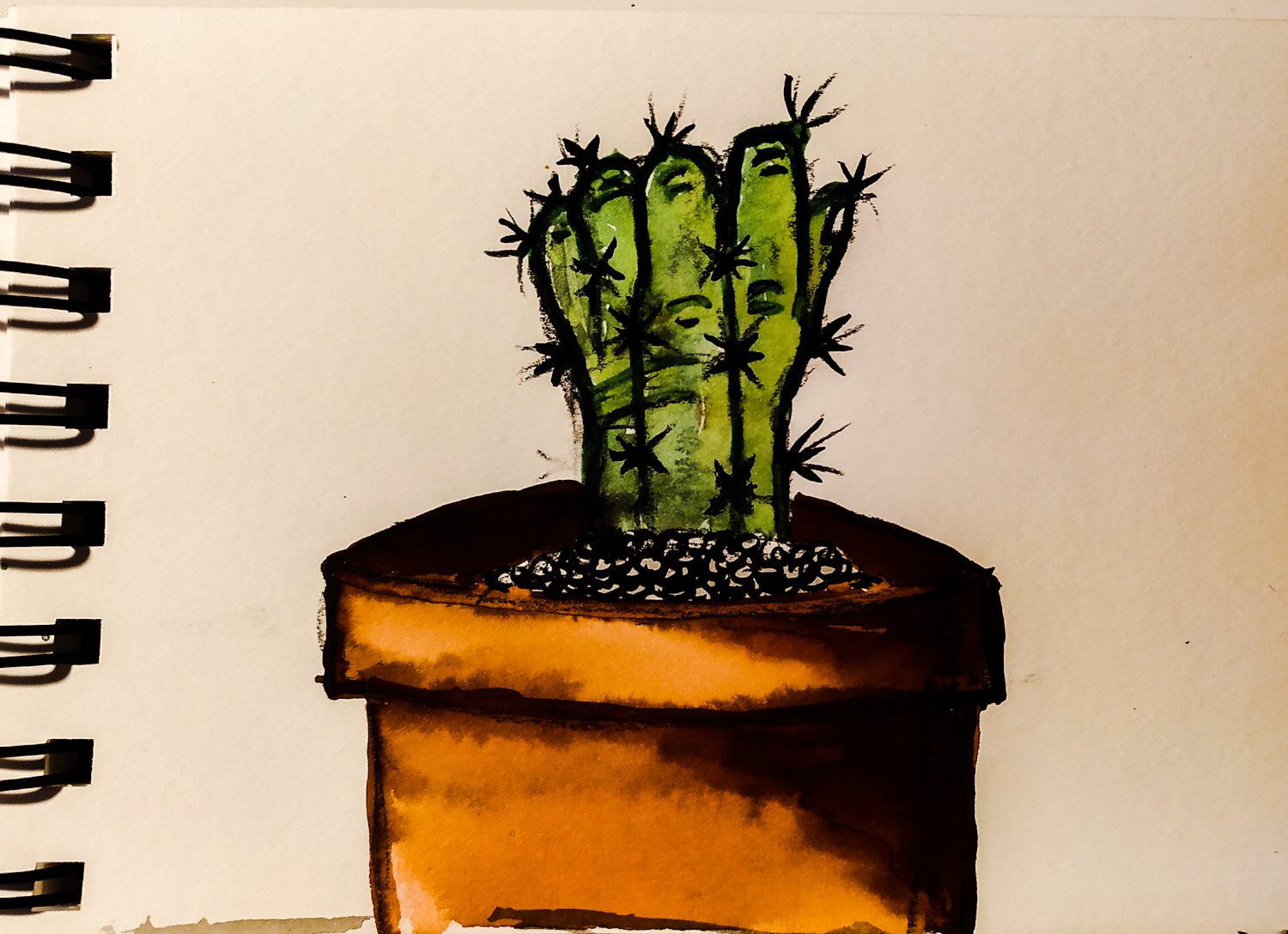A detailed and intricate artwork, likely a painting or drawing, is depicted on a page of a spiral-bound notebook. The focal point is a green cactus adorned with numerous sharp spikes, residing in a notably oversized terra cotta pot. The pot, with its rustic hue and coarse texture, occupies a significant portion of the composition, contrasting with the smaller size of the cactus, which fills less than a third of the pot. The artist has skillfully employed a mixture of colors to highlight the intricacies of the coarse potting mixture. Additionally, the use of shadows enhances the depth and three-dimensionality of the scene, adding a realistic touch to the artwork.